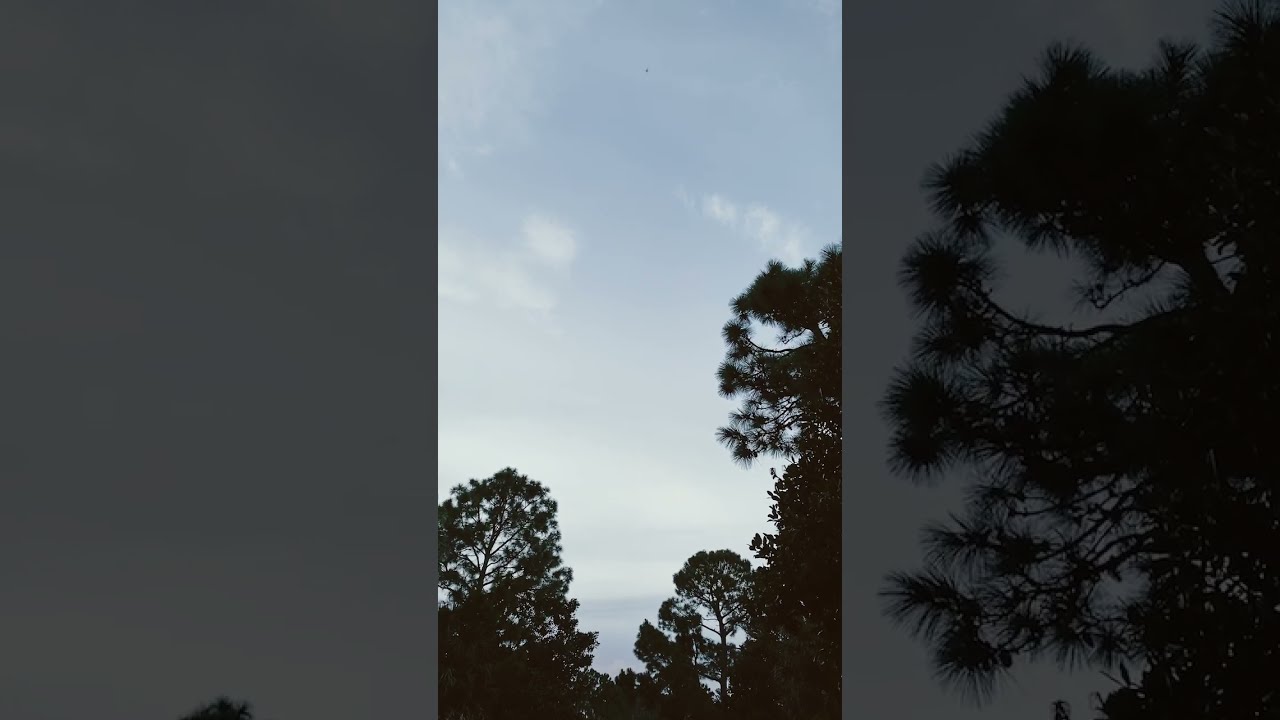The image captures the silhouette of several tall trees, possibly ferns and needle-like pine trees, extending their treetops into a cloudy sky. The photo appears to have been taken with a cell phone and is oriented vertically, nestled within a larger, landscape-oriented frame. To the left and right of the main vertical image, there are darkened close-ups of the same scene, adding a sense of depth and focus to the central composition. In the background, the sky is light blue with patches of gray and white clouds, including a small, distinct puffy cloud on the right. A crescent moon is delicately visible between the branches of the far-right tree. The trees, silhouetted in shadow, resemble the shape of broccoli, with slender trunks and dense, branching tops. At the base of the scene, an indistinct area could either be a body of water or an unusually flat-looking cloud. The tranquil composition emphasizes the contrast between the dark tree silhouettes and the ethereal sky above.